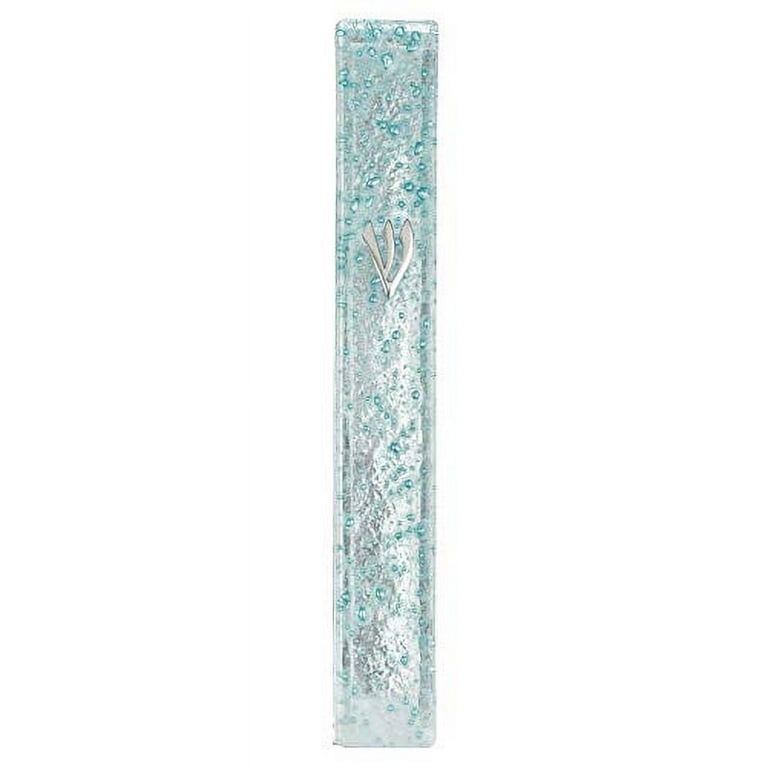In the image, against a plain white background, there is a long, rectangular object with a portrait layout, meaning it's much taller than it is wide. The object appears translucent, possibly made of glass or plastic, and is tinged with shades of turquoise or seafoam green. Scattered across it are small, bubble-like markings that add texture to the otherwise clear material. About 30-40% down from the top, there's a prominent silver "W" logo or design element attached to it, which could be metallic or reflective. Additionally, there is a three-pronged, sword-like engraving around this "W" logo. The entire object resembles a flat, tube-like container or possibly a roller stick, with both ends sealed, evoking the appearance of packaging for a squeezable product. While its exact purpose remains ambiguous, it evokes comparisons to items like a squeezable tube of lotion or gel.